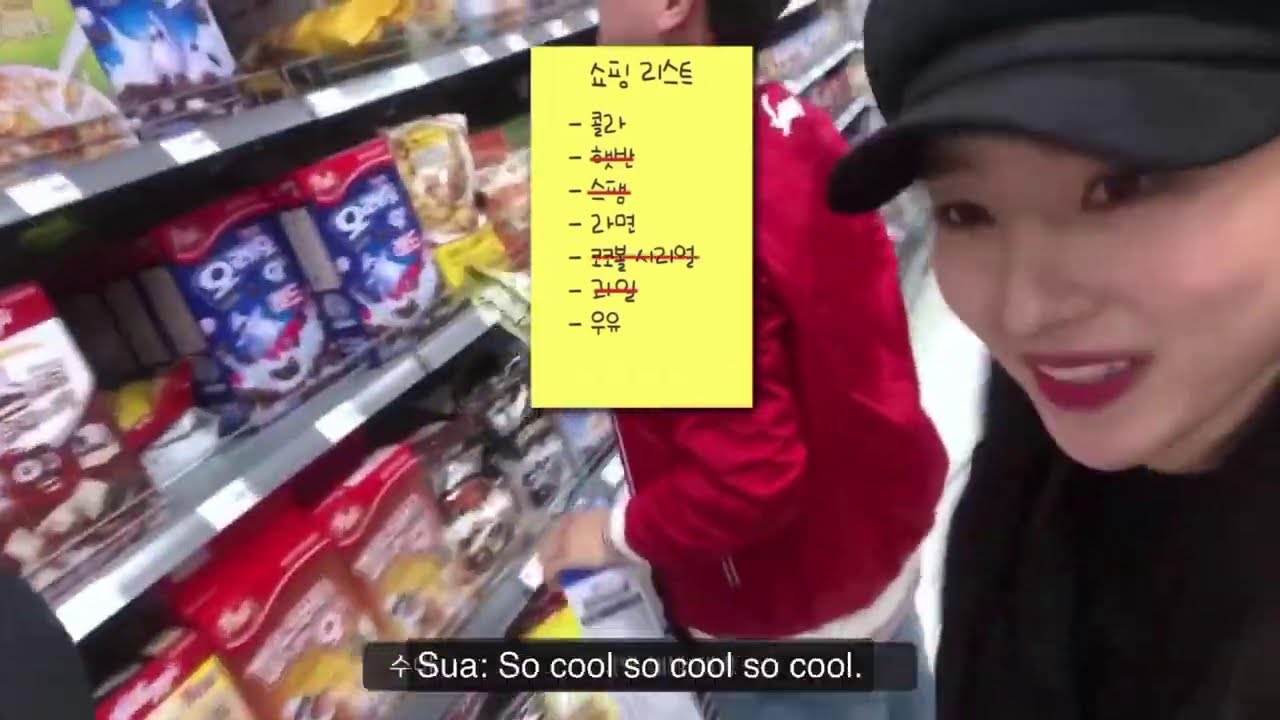The image appears to be a screenshot from a video taken inside a supermarket. At the center of the image, slightly above the middle, there is a yellow shopping list with seven black symbols, some of which are crossed out with red lines. Above the list is a word made up of symbols, possibly Korean text. At the bottom of the list, in a brown bar with white letters, it reads "SUA: so cool, so cool, so cool." 

In the left portion of the image, there is a man wearing a red coat and blue jeans. His black hair is barely visible as his head is cut off by the frame. He appears to be inspecting items on a shelf, which could be cereal boxes or chips, although the image is slightly out of focus in this area. To the right side of the image, a woman with red lipstick, dressed in a black top and black hat, holds the camera and has a half-smile on her face. The setting overall is inside a grocery store with various food items on the shelves.

Predominant colors in the image include black, red, yellow, tan, orange, green, and white.